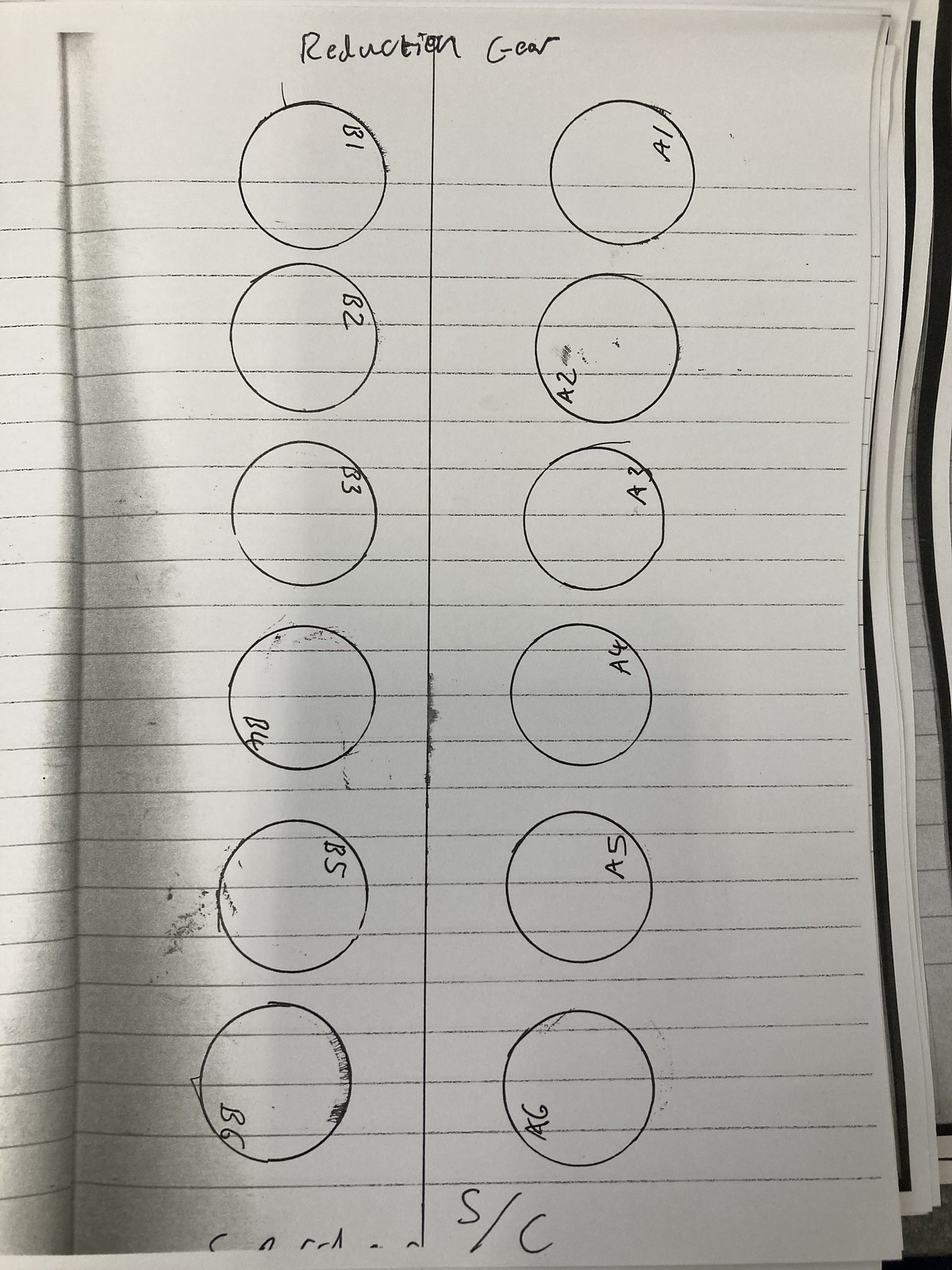The image showcases a detailed photograph of a lined notebook paper, appearing to be part of a composition book that has been folded open. Other pages are visible in the background, and the right side of the open page seems ripply, possibly due to water damage, a ding, or the angle of the camera.

The focal page is distinguished by its evenly spaced, horizontal grayish lines. A vertical line, meticulously drawn with a ruler or straight edge, bisects the page. Additionally, two neatly traced columns of circles are present, indicating the use of a compass or protractor.

At the top, within the wide white margin before the lines start, is a handwritten heading, which reads something like "reduction," "goal," or possibly "gear," although the exact word is unclear.

The left column contains six labeled circles: B1, B2, B3, B4, B5, and B6. The right column mirrors this with six circles labeled A1, A2, A3, A4, A5, and A6. Each alphanumeric label is placed within its respective circle, although the positioning varies:

- **Left Column:**
  - B1, B2, B3: Top right quadrant (written sideways)
  - B4: Bottom left quadrant
  - B5: Top right quadrant
  - B6: Bottom left quadrant

- **Right Column:**
  - A1: Top right quadrant
  - A2: Bottom left quadrant
  - A3: Top right quadrant
  - A4 and A5: Top right quadrant 
  - A6: Bottom left quadrant

Toward the bottom of the page is a word written in pencil, though partially cropped out of the frame, it seems to start with an "S." Adjacent to this word, there appears to be another notation, “S / C,” but the exact details are cut off.